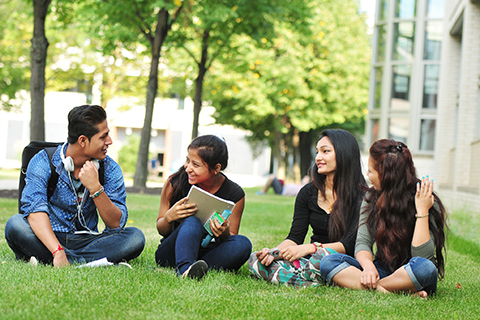This vibrant photo captures a diverse group of four students sitting on green grass outside a large building with many windows, framed by several green-leaved trees. The students appear to be enjoying a casual, sunny day, as they all have genuine smiles and engage with one another in conversation. On the left, a young man with dark brown skin is wearing a blue button-down shirt, jeans, and has white headphones around his neck. He also sports a bracelet and has a black backpack on his back. Sitting next to him is a woman in a black tank top and black stretch pants, holding a notebook and a blue-handled object that seems to be a juice box. She, like the rest, is smiling warmly. The woman on her other side is wearing a black three-quarter length sleeve shirt and colorful pants, her gaze directed to the left with a cheerful expression. On the far right, there is a woman with long, dark brown hair, partially clipped back with hints of red highlights. She’s dressed in a gray three-quarter length sleeve shirt and capri jean pants. All four students share dark brown hair and skin, and their relaxed postures reflect a moment of joyful camaraderie on a picturesque day.